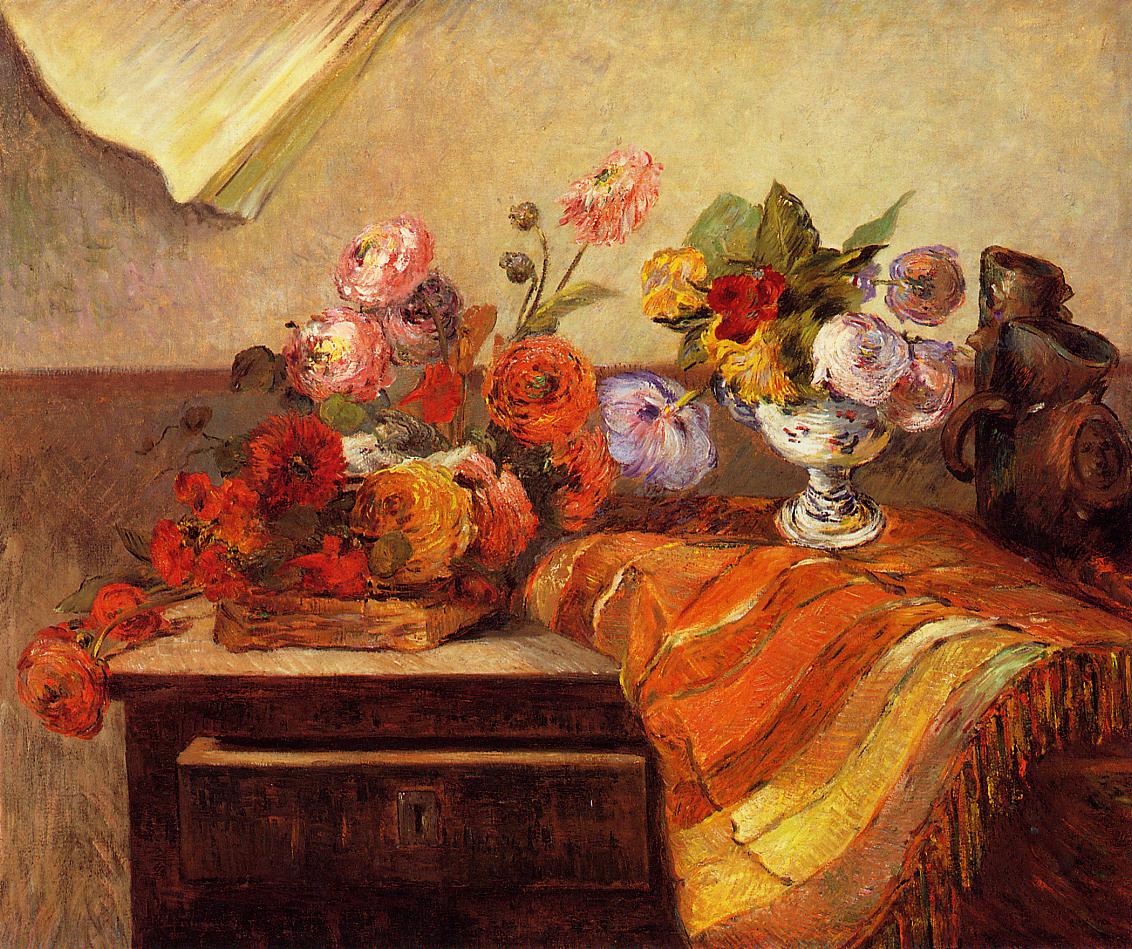This painting evokes the Impressionist style reminiscent of Van Gogh, featuring a vibrant and colorful arrangement of artificial flowers adorning a brown wooden nightstand with a drawer slightly open. The flowers, in hues of red, orange, pink, and yellow, overflow from a silver bowl and a small basket. An orange cloth with red, yellow, and white stripes drapes over the nightstand, enhancing the warm and cozy atmosphere. The background showcases a two-toned wall, lighter tan on top and darker brown on the bottom, with brushstrokes visible in the lighting, contributing to the overall texture. A few flowers extend over the edge of the table, adding a dynamic element, while dark vases stand prominently on the right. The scene exudes a serene stillness, focusing solely on the floral arrangement in a domestic setting, possibly a kitchen or bedroom.